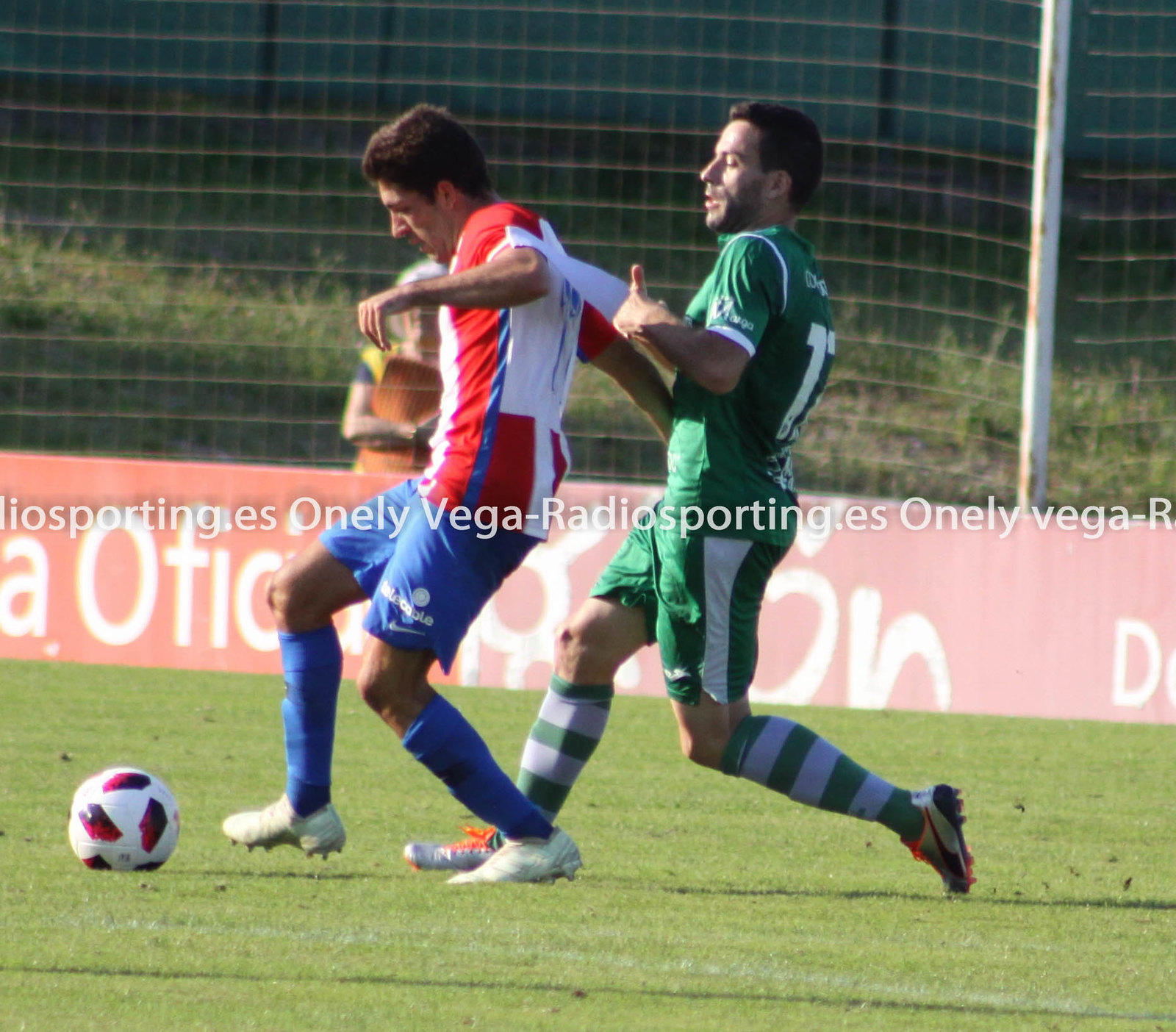In the image, two soccer players are intensely vying for control of a soccer ball situated at the bottom left. The player on the left, wearing a red and white vertically striped shirt with sky blue shorts above the knee, positions his foot just behind the ball. His attire also includes long blue socks that reach below the knee and trainers featuring blue, dark blue, and white colors. The player on the right is dressed in a green top and green shorts with a white stripe, complemented by horizontally striped white and green socks that reach just below the knee and multicolored shoes in white and blue.

The photo is overlaid with white text across the center, reading "OneLeagueVega-RadioSporting," which repeats horizontally from left to right. In the background, a soccer net is visible, indicating the late time of day as the sun shines brightly. A spectator stands behind a protective barrier behind the player in the red and white uniform. The spectator is partially obscured by the barrier. Behind the net stretches a grassy embankment that angles upward from the field. There are no other players visible on the field, making the focus solely on the two competitors.